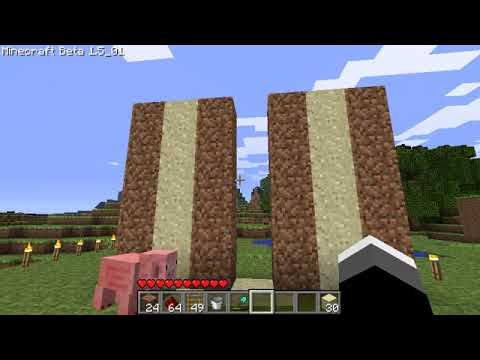This image captures a scene from the Minecraft Beta 1.5-01 game. In the top-left corner of the screen, the game's version can be seen. Dominating the upper part of the scene is a brick wall with three vertical blue streams resembling doors. In front of this wall, a green grassy area extends across the foreground. There is also a notable hole in the ground, occupied by the player character who appears ready to dig, holding a ladder in their right hand and aiming a crosshair at the ground. 

Additional elements include wooden railings and brown structures emerging from the ground, suggesting a diverse environment. On the right, a waterfall flows towards the player, and dirt is visible around this water feature. At the bottom of the screen, the HUD displays the player's health with 12 red hearts. The item bar contains various tools and materials including wood, redstone, a bucket, a ladder, a shovel, and sand, with corresponding counts of 24, 64, and 49 in different squares.